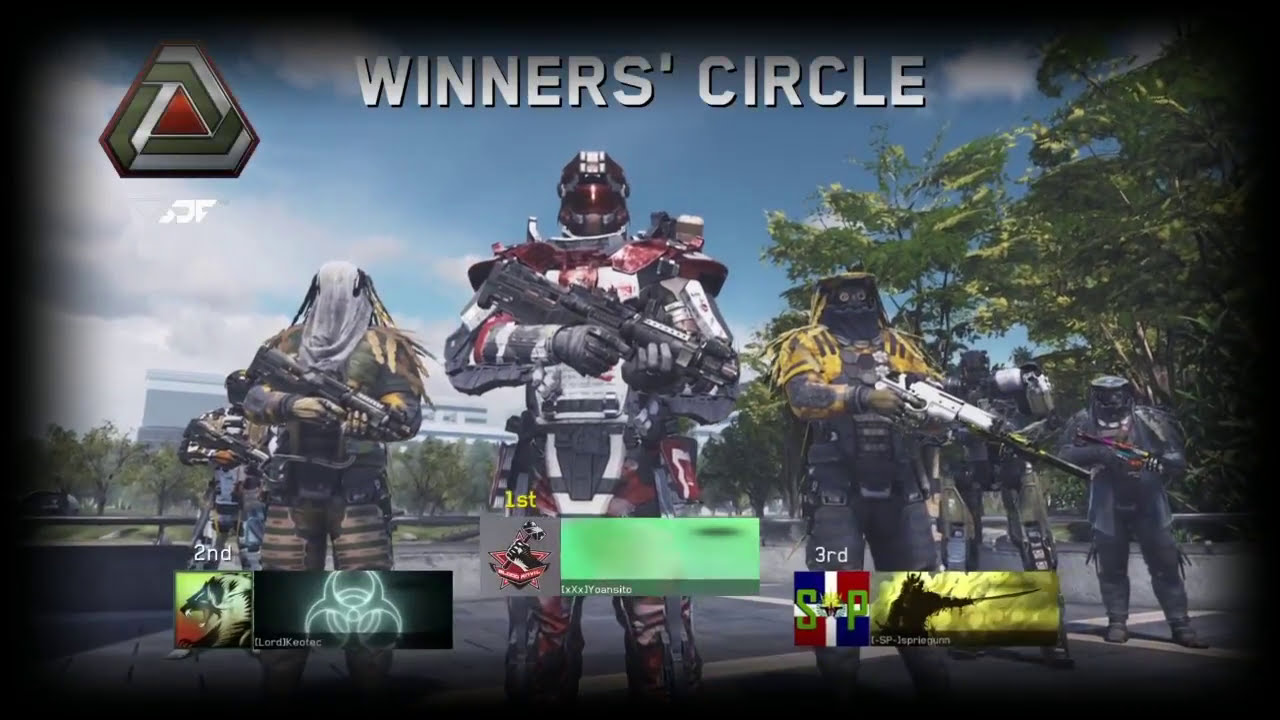The image portrays a detailed end-game screen from a shooter video game, highlighting the "Winner's Circle." Dominating the scene are six digital soldiers in a meticulous formation. At the forefront, three prominent characters signify the top finishers: first place is the central figure adorned in white, black, and red armor with a helmet, clutching a long rifle; flanked by second place on the left in traditional army camouflage; and third place on the right, also in camo but with a distinct yellowish theme. 

Beneath each of the top three are their gamer tags, profile pictures, and banners indicating their ranks. The backdrop features a cement ground, suggestive of a sidewalk or road, and a landscape with deciduous trees and a faint cityscape under a cloudy blue sky. Additional digital soldiers align in the rear, equipped with futuristic mech-like armor and weaponry. Encasing the scene, a triangular logo with white, green, and reddish-orange hues embellishes the top-left corner, while the text "Winner's Circle" is prominently displayed at the top in white font. The carefully arranged scene emphasizes the victorious players within the immersive game environment.